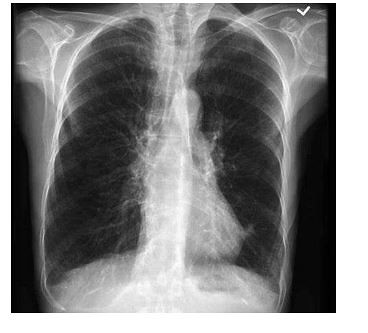This image showcases a detailed x-ray of a person's torso, set against a black background. The shoulders are prominently visible at the top left and right corners, with the spine running down the center, appearing white against the otherwise dark chest and abdominal regions. The rib cage is visible, characterized by horizontal lines indicating the ribs, with black spaces between each one. Notably, there is a cloudy white mark in the bottom right side of the image, near the spine, within the abdominal area. Additionally, a small white checkmark can be observed near the shoulder in the upper right-hand corner. Despite this clouded area, the x-ray remains relatively clear overall.